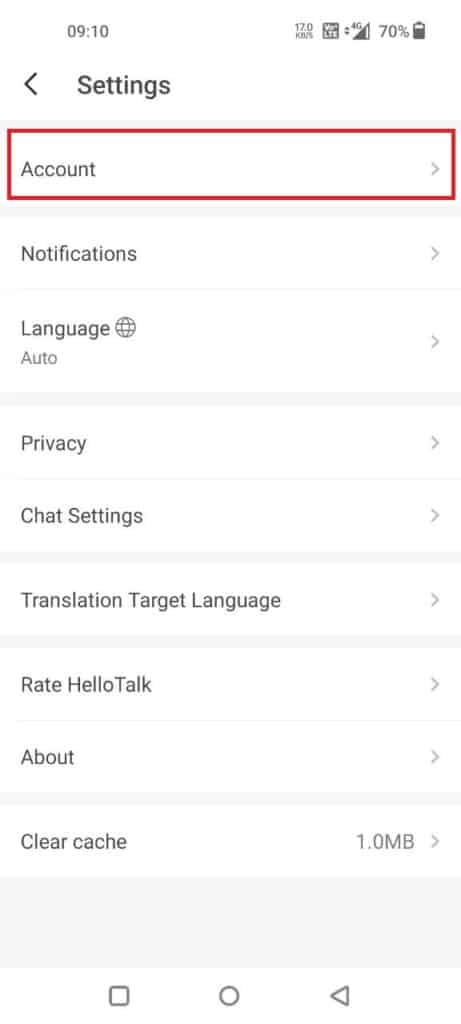The image depicts a screenshot of a smartphone displaying the settings menu. In the top-left corner of the screen, the clock shows the time as 09:10. On the top-right, there are icons indicating the device's signal strength and battery level, which is currently at 70%.

Below this, the title "Settings" is prominently displayed in grey. A vertical list of settings options follows, including "Accounts," "Notifications," "Language," "Privacy," "Chat Settings," "Translation," "Target Language," "Rate," "Hello," "Talk," "About," and "Clear Cache." Each option is accompanied by a small arrow on the right side, indicating that they can be expanded for more details. Notably, the "Accounts" option is highlighted with a red rectangular box drawn around it.

The "Language" option includes an icon resembling a globe and the word "Auto," suggesting automatic language settings. Finally, at the bottom of the screen are three shapes: a square, a circle, and a rectangle, whose significance is unclear but are prominently displayed as part of the smartphone's interface.